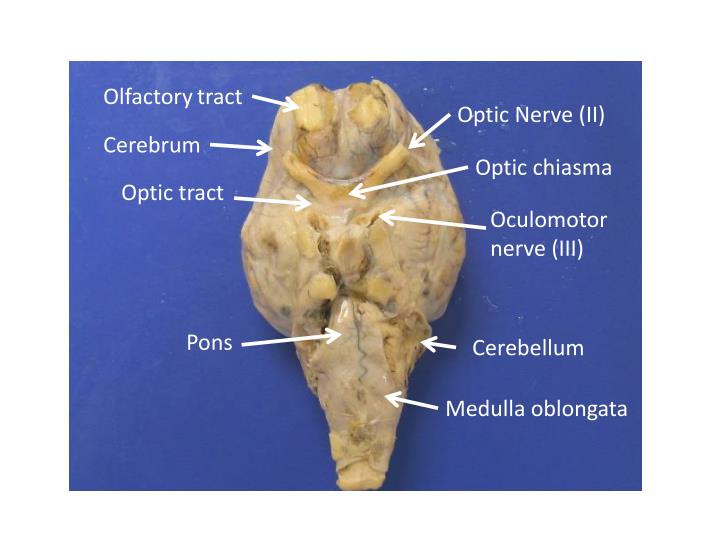This photograph features a detailed medical diagram of a brain, potentially from an animal or human. The brain, appearing yellowish or pale, is meticulously laid out on a light blue background. Various parts are labeled in white text, with arrows indicating specific regions. At the top left corner, the olfactory tract is identified, followed by the cerebrum, optic tract, and pons. On the right side, from top to bottom, are the optic nerve, optic chiasma, oculomotor nerve, cerebellum, and medulla oblongata. Each label in the image is clearly marked with directional arrows to aid in identifying the precise locations of these anatomical features.